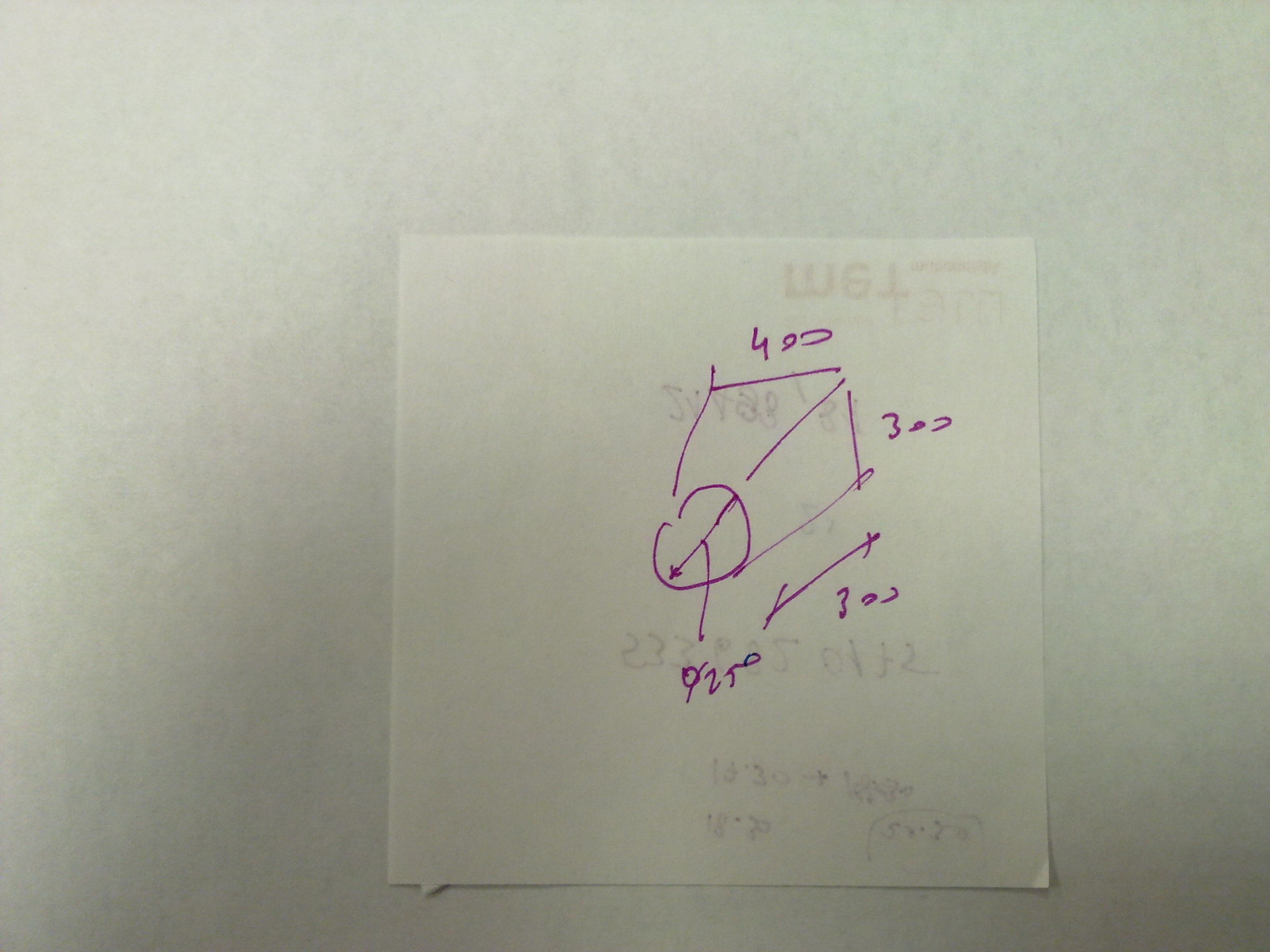A piece of paper is shown with handwritten notes in purple ink, likely belonging to a high school or junior high student. The notes detail a geometry problem featuring a truncated pyramid-like shape, with a circular top surface. Various dimensions are labeled: the diameter of the circular top is marked as 250 units, the height of the shape is 300 units, and the base dimensions are annotated as 400 by 300 units. Additionally, the translucency of the paper reveals some non-geometry notes on the reverse side, suggesting a mix of mathematical exercises. The paper serves as a candid glimpse into a student's effort to solve complex geometry problems.